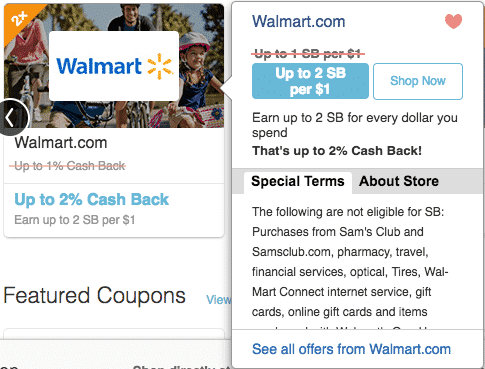This is a screenshot of a pop-up menu on Walmart's website. The pop-up menu has a white background. In the upper left corner, it features "walmart.com" written in blue font. In the upper right corner, there is a red heart icon. Below the heart icon, the text "up to 1 SB per dollar" is crossed out in red. Underneath this, a light blue rectangle contains the text "up to 2 SB per dollar." Adjacent to this, on the right, is a white rectangular button with blue font that reads "shop now."

In black font below these elements, the text explains: "Earn up to 2 SB for every dollar you spend, that's up to 2% cash back." Directly beneath this, a gray bar displays the selectable options "special terms" (currently selected) and "about store."

Under the "special terms" section, the text specifies that the following purchases are not eligible for SB:
- Purchases from Sam's Club and samsclub.com
- Pharmacy
- Travel
- Financial services
- Optical
- Tires
- Walmart Connected Internet Service
- Gift cards
- Online gift cards

The text cuts off here, requiring scrolling down to read more. At the bottom of the pop-up, there is a white rectangular button with blue font that says "see all offers from walmart.com."